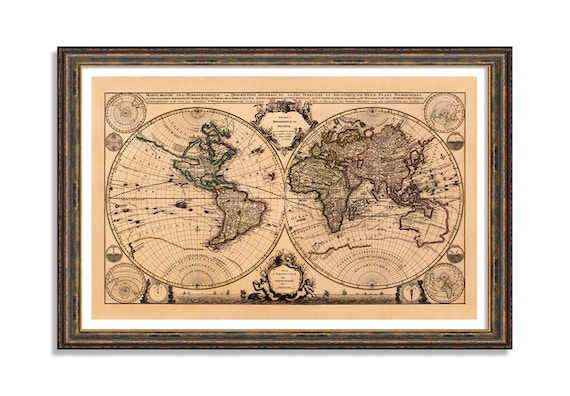This framed, horizontal, rectangular image is a vintage reproduction of an old world map. The map is divided into two hemispheres, displayed side by side within circles, and is set against a brown background. The continents on the map are darker colored and outlined in shades of dark green, red, and yellow, giving them an aged and exploratory appearance, consistent with maps from the 18th or 19th centuries.

The map is meticulously detailed with lines of longitude and latitude, and contains numerous embellishments and writing, though the text is too small to read clearly. The continents are depicted with less precision compared to modern maps, showcasing odd and incomplete shapes, particularly in areas like North America and Canada, which suggests that the map was created before the complete exploration of these regions. 

The illustration is matted with a white border and encased in a wooden frame. Additional decorative elements include a coat of arms situated centrally between the two hemispheres and another at the top, with circular embellishments in each corner of the map. Despite the imperfect representation of landmasses like Antarctica and Australia, the map provides a fascinating historical insight into the world as it was known at the time of its creation.